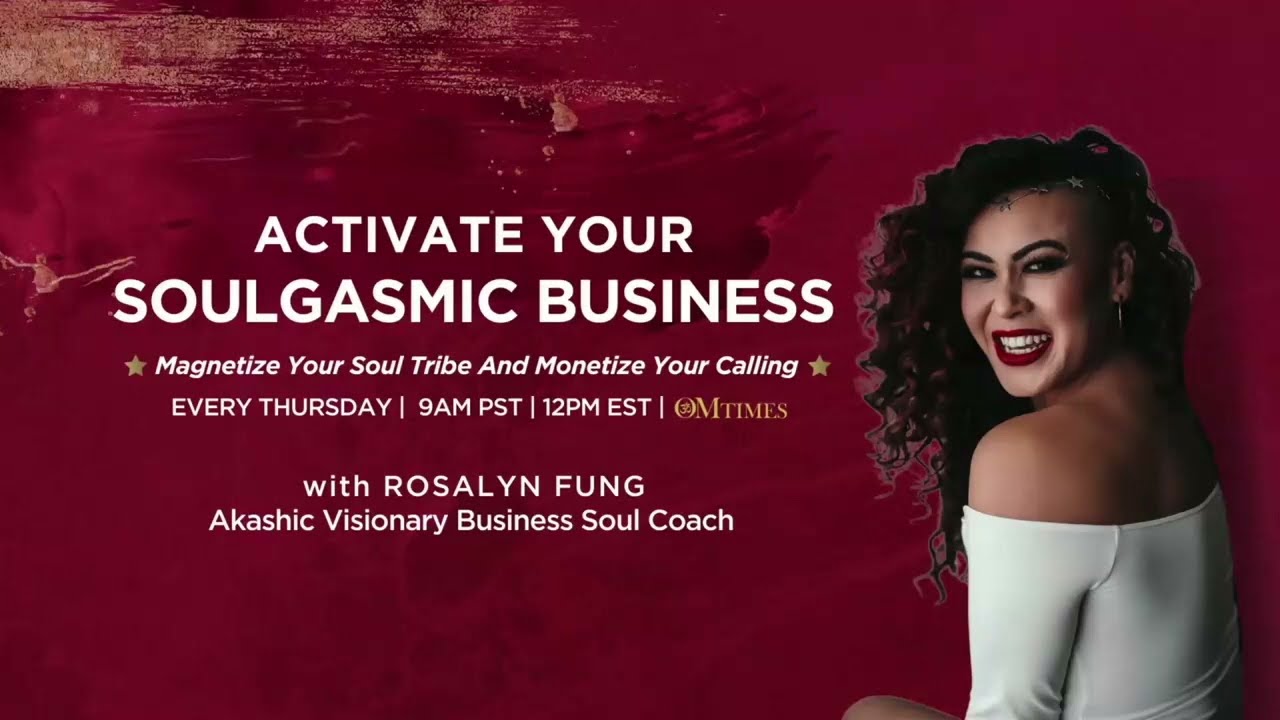In this striking advertisement featuring a dynamic business coach, Rosalind Fung, a confident Hispanic woman commands attention on the right side of the image. She turns her head back slightly to the right, her gaze forward, exuding poise and charisma. Her dark, curly hair cascades down to just below her chest, with a stylish part to the left. Her vibrant smile, accentuated by bright red lipstick and gleaming white teeth, complements her expressive dark eyebrows. She dons a sleek white suit that elegantly frames her shoulders and upper back, paired with a noticeable earring in her left ear.

The maroon, almost magenta, background provides a bold canvas with brush strokes of the same color on the upper left, creating a textured and dynamic effect. Central to the image is the compelling message in clean white lettering: "Activate your soulgasmic business. Magnetize your soul tribe and monetize your calling." Each phrase is flanked by delicate white stars, adding a touch of whimsy and emphasis. Below, it states the timing of her offering: "Every Thursday, 9 a.m. PST, 12 p.m. EST," suggesting a regular event, likely a podcast or webinar. Further details in gold lettering identify Rosalind Fung as the "Akashic Visionary Business Soul Coach," inviting viewers to engage with her unique and magnetic guidance.